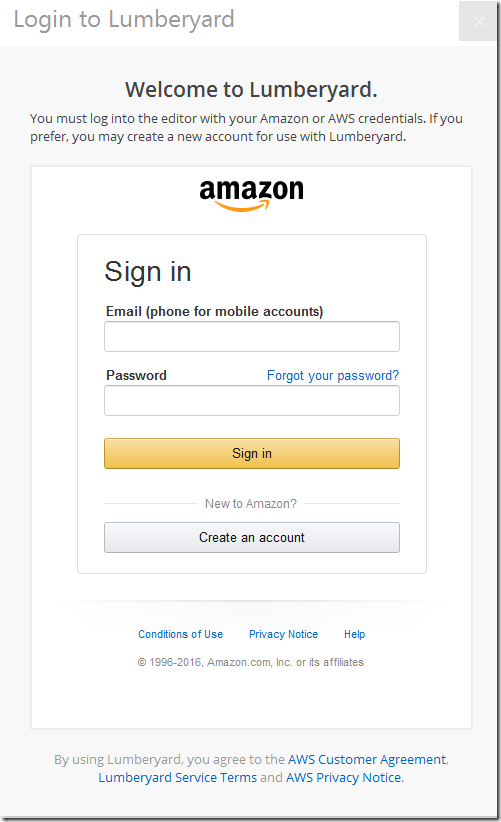The image displays a login page for Lumberyard, prominently featuring the Amazon logo at the top. Below the logo, the page greets users with "Welcome to Lumberyard" and instructs them to log in using their Amazon or AWS credentials. A white input box follows for entering login details. The first field is labeled "Email or mobile phone number for mobile accounts," followed by a field for the password, which is accompanied by a blue hyperlink that reads "Forgot your password?" Beneath these input fields is a large, rectangular orange button labeled "Sign in."

Further down, the page addresses new users with the text "New to Amazon?" and provides a large gray button labeled "Create an account." At the very bottom of the page, several links are displayed: "Conditions of Use," "Privacy Notice," and "Help." The footer concludes with the text, "1996-2016, amazon.com, Inc. or its affiliates."